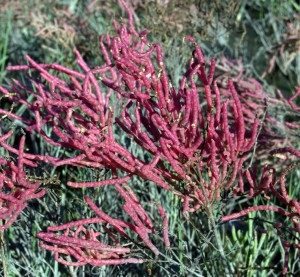The photograph features an intriguing plant adorned with long, cylindrical, reddish-colored growths that resemble chili peppers or wiry flowers. These striking red elements have a finger-like appearance, curving in various directions, and create a vivid contrast against the surrounding greenery. Abundant dark green stems form the backdrop, transitioning to lighter green shades toward the foreground. The plant is accompanied by other greeneries, which appear slightly brownish and dry, highlighting the lush vibrancy of the featured plant's red and green hues.